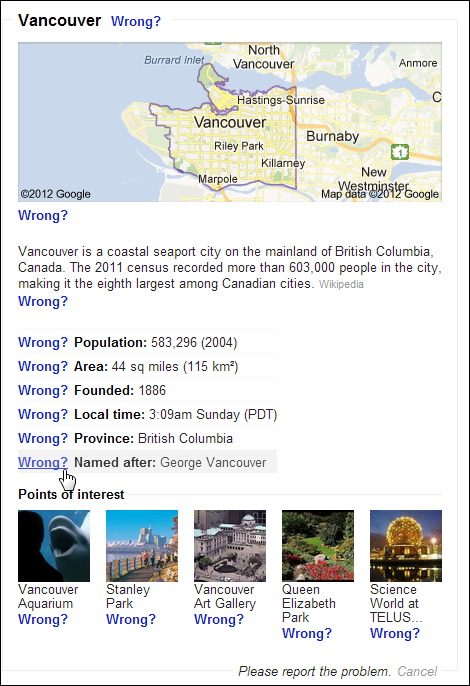This vertically oriented screenshot features a detailed layout of information about Vancouver, bordered by a black frame. The primary background color is white. At the top left corner, the word "Vancouver" is prominently displayed with a peaceful blue typographic style, abruptly followed by "wrong?" scattered in blue text throughout the entire image, raising an inquiry into the accuracy of the content presented.

The upper section showcases a map of Vancouver, providing a geographical context. Below the map, there is a comprehensive description of Vancouver, framed by the question "wrong?" prominently positioned at the lower left corner. The textual content details that Vancouver is a coastal seaport city on the mainland of British Columbia, Canada, with a 2011 census population of over 603,000, making it the eighth largest city in Canada. Each piece of information, such as population, area, founding date, local time, province, and the city's namesake, is prefaced with the word "wrong," creating a repetitive questioning motif.

Towards the bottom of the image, five colored photograph icons are laid out in a square formation under the heading "Points of Interest." These thumbnails represent notable locations in Vancouver: Vancouver Aquarium, Stanley Park, Vancouver Art Gallery, Queen Elizabeth Park, and Science World at TELUS.

The bottom right-hand corner within the black border presents the options "Please report the problem" and "Cancel," inviting user interactions to address perceived inaccuracies. The captured layout portrays a dense yet meticulous compilation of Vancouver's geographical and cultural attributes, juxtaposed with an overarching skepticism embodied by the frequent "wrong?" text.